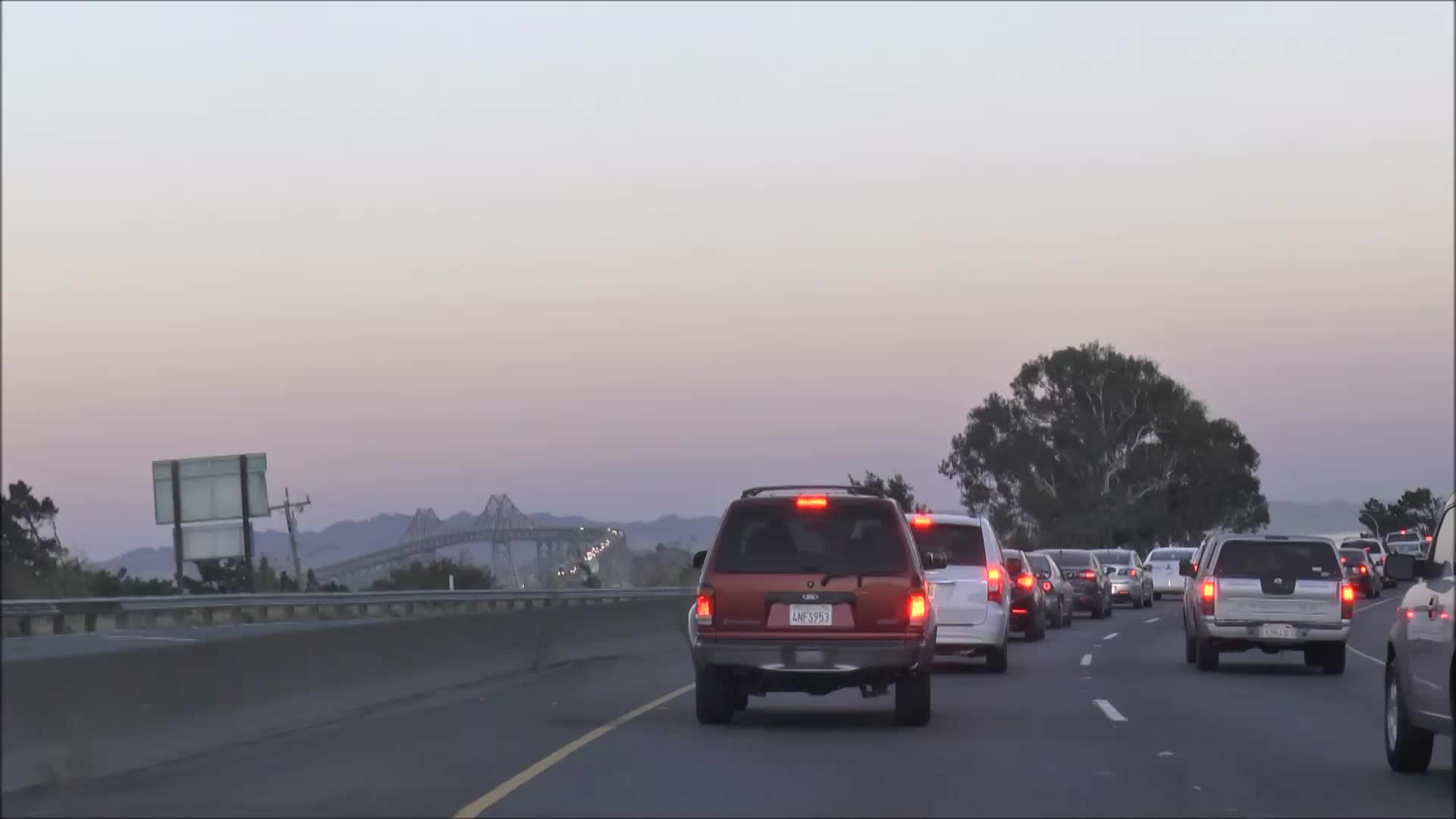This wide-angle photograph captures a congested highway scene from the perspective of a driver in the left-hand lane of a two-lane road. The view showcases bumper-to-bumper traffic as the road curves to the right. Every visible vehicle ahead has its brake lights illuminated, indicating a slowdown or complete stop. The car directly in front is an SUV with the license plate 4NF5953. Near the curve, a tree stands tall, creating a natural landmark for the area. In the background, on the left-hand side, a bridge looms, with headlights of oncoming vehicles descending on the opposite side. This suggests that the traffic jam is occurring just before the bridge, often a common bottleneck. The photograph also captures the yellow shoulder lane to the left and the dividing line between the left and right lanes of the highway on the right, adding to the detailed depiction of the scene.